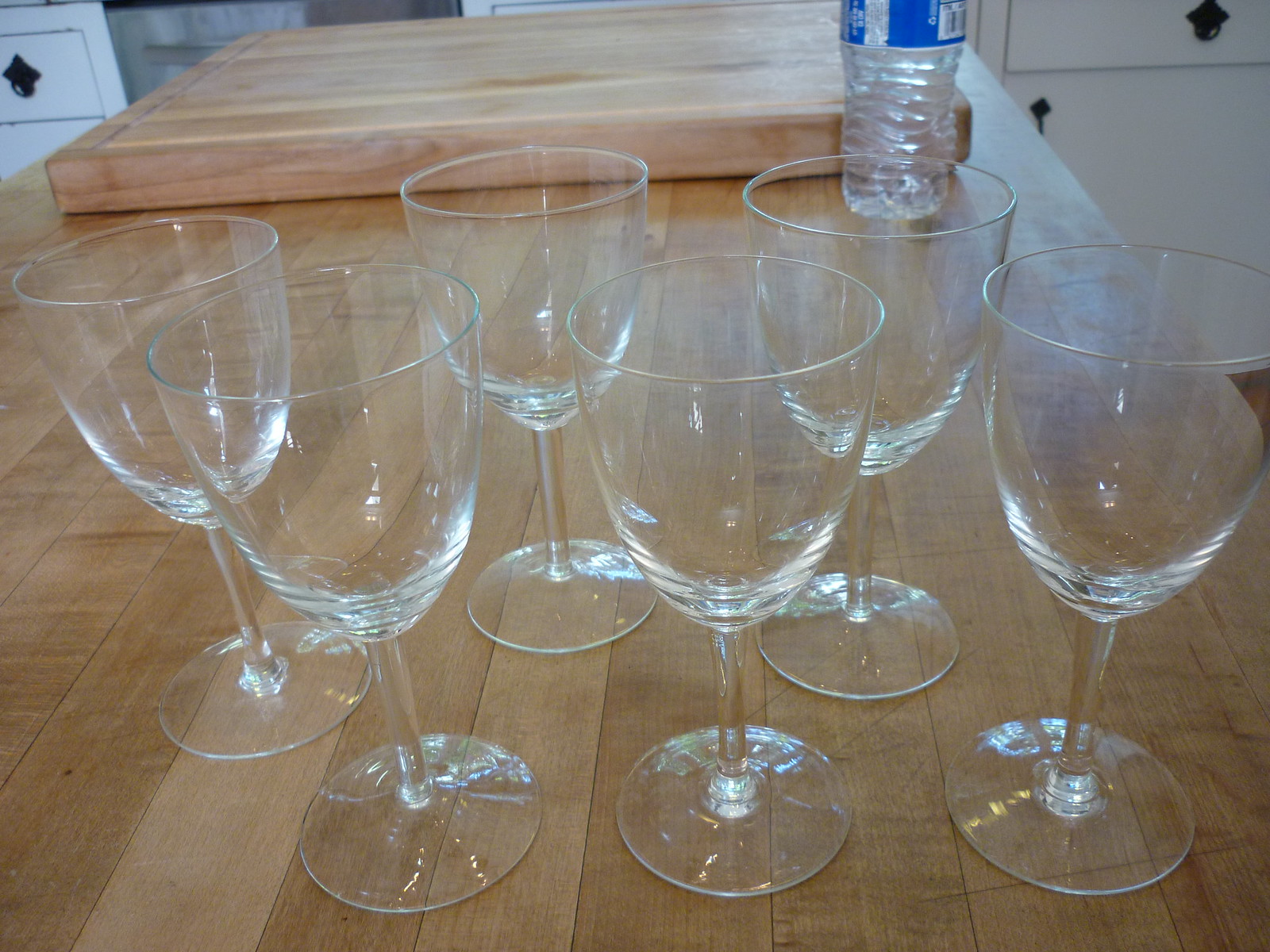The detailed caption: 

This image captures a close-up view of six clear, empty wine glasses arranged in two neat rows of three on a light brown wooden countertop. The glasses have medium-length stems and slightly wide, tulip-shaped bowls, with their reflective surfaces suggesting natural lighting. The countertop extends towards the back where a large, solid wood cutting board, about an inch thick, is positioned. In front of the cutting board, a partially visible bottled water with a blue label stands, distorting slightly due to the lens angle. The background features white kitchen cabinets with black handles and knobs, alongside what appears to be the door of a dark gray oven. The composition emphasizes the reflective clarity of the glasses against the warmly lit kitchen environment.